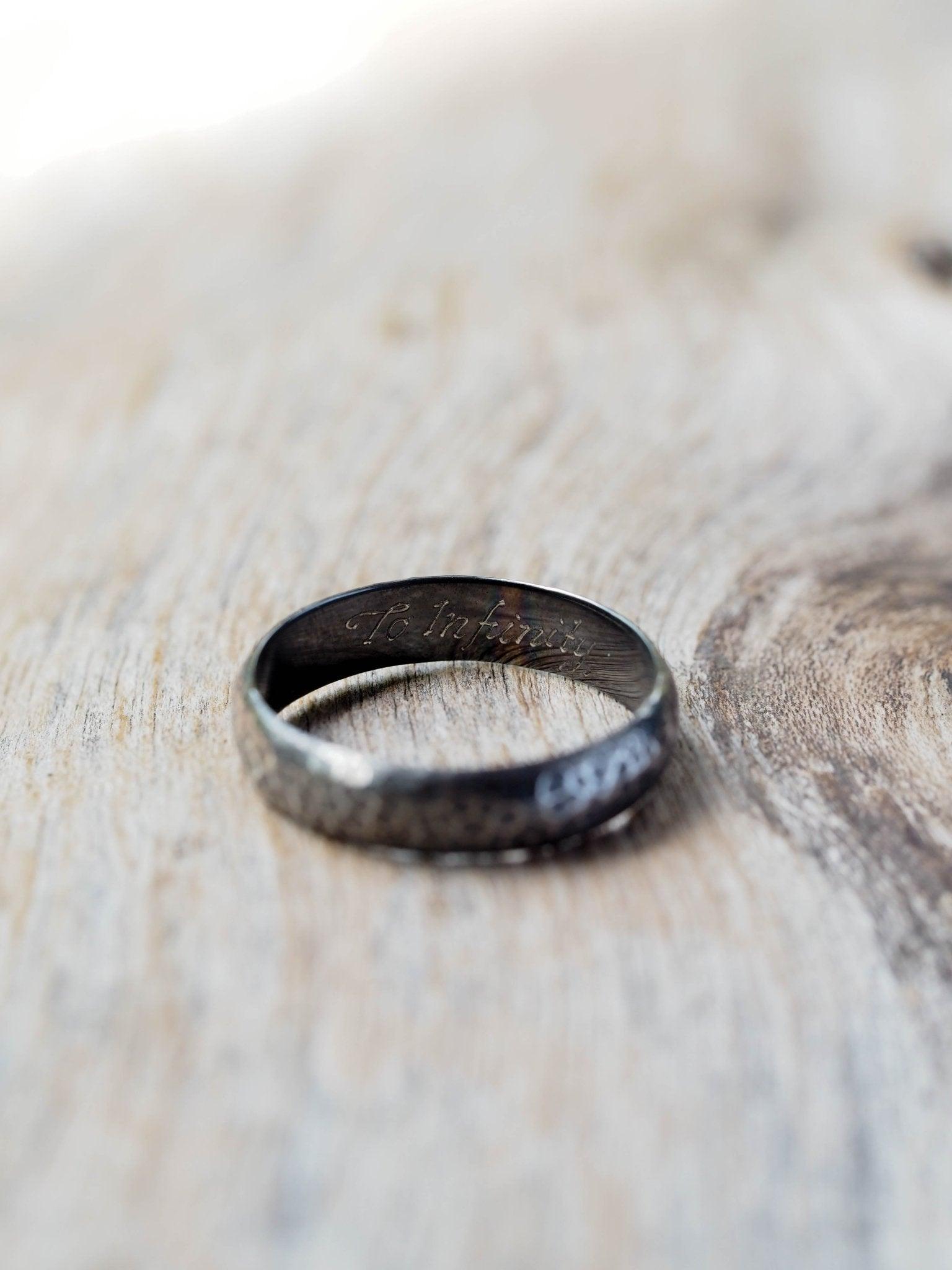This close-up photograph features an aged and tarnished silver ring with a hammered texture on the outside. The ring, which resembles a wedding band, displays an engraving on its inner surface that reads "to infinity" in a cursive script. The piece is positioned on a weathered gray wooden surface, characterized by a fine grain and a noticeable knot on the right side. The lighting, soft and almost dreamlike, comes from the left, casting a shadow to the right. The top and bottom parts of the image are blurred, adding to the focus on the ring and the detailed wood grain underneath. The ring's old, unpolished appearance contributes to its rustic charm, reminiscent of a cherished piece of hand-forged jewelry.